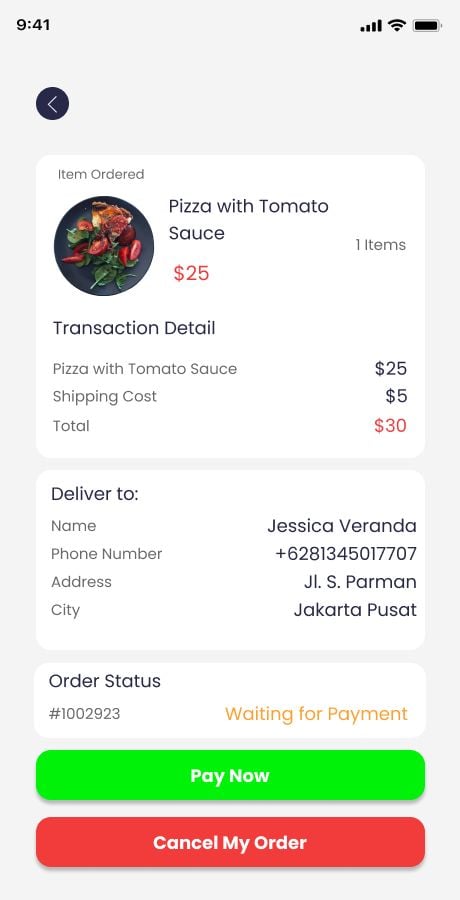The image depicts an order page displayed on a mobile app with a white background. 

At the top left corner, the time is shown as 9:41, and on the top right, there are icons indicating cell signal strength, Wi-Fi connection, and battery level, which is approximately 96-97%. Below the time on the top left, there is a black circle with a white arrow, indicating a button to go back to the previous screen.

The center of the image features three white boxes stacked vertically:

1. The first box is titled "Items Ordered." It lists "Pizza with Tomato Sauce" as the ordered item, priced at $25. A breakdown of the transaction details follows: "Pizza with Tomato Sauce - $25", "Shipping costs - $5", totaling "$30."

2. The second box is labeled "Deliver To" and contains the recipient's details: name (Jessica Veranda), phone number, address (JLS Parman), and city (Jakarta Pusat).

3. The third box provides information about the order, showing the "Order Number" and "Order Status." The status is "Waiting for Payment," highlighted in orange. Below this status, there are two buttons: a green "Pay Now" button and a red "Cancel My Order" button.

The layout and design of the page are straightforward, allowing the user to easily view and manage their order details.